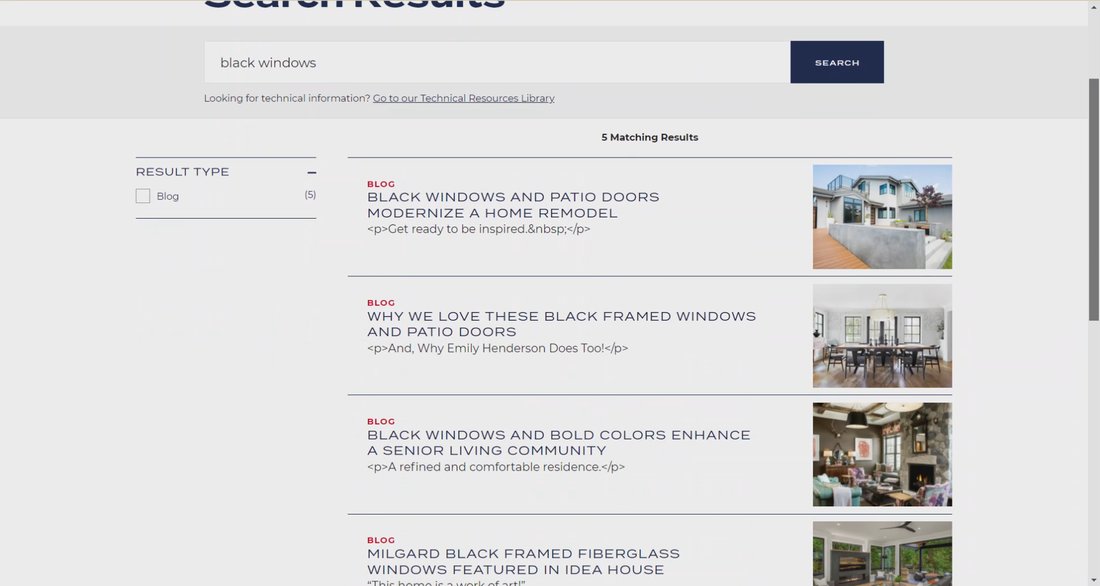"During a search for black windows, four matching results were prominent, each offering a unique perspective on the aesthetic appeal of black-framed windows in various settings. The first result features an image of a white house or potentially a houseboat by a canal, highlighting a blog that says, 'Black windows and patio doors modernize a home remodel. Get ready to be inspired.' This picture emphasizes the elegant contrast created by black windows and patio doors set against the light exterior of the house. 

The second blog result is titled, 'Why we love the black framed windows and patio doors,' though the text cuts off before fully revealing why Emily Harrison appreciates them. The accompanying image captures a spacious dining room adorned with hardwood floors. The walls are painted white, but the standout feature is the large, black-framed windows at the room's end, which frame the view outside with chic black panes.

Another blog discusses how 'Black windows and bold colors enhance a senior living community,' portraying it as a refined and comfortable place of residence. The image showcases the senior living community adorned with black windows, which sharply contrast with the surrounding colorful structures, adding a modern touch to the overall design.

The last result, though cut off, mentions a 'Milgard black-framed fiberglass window featured in Idea House,' but lacks an image to provide further context. Despite this, it tees up intrigue about the role of black windows in innovative home design."